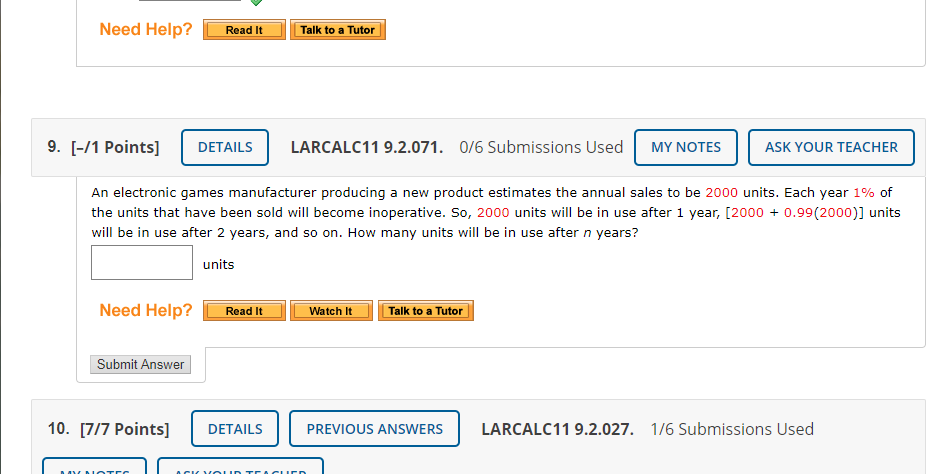This is a partial screenshot from an educational website with some cropped details. The main content prominently displays "9" at the beginning, indicating the question number. In brackets, it states "[1 point]," denoting the value of the question. Below this, there is a grey bar featuring several buttons, including "Details," "My Notes," and "Ask Your Teacher." The username is visible, along with a note that says "0 out of 6 submissions used."

Directly beneath, the text box contains a math problem related to an electronic games manufacturer. The problem outlines that the company estimates annual sales of 2,000 units, with 1% of the sold units becoming inoperative each year. The description continues with a mathematical expression to explain the calculation: "2,000 units will be in use after one year (2000 × 0.99). After two years, it will be (2000 × 0.99^2), and so on." The question seeks to find the number of units that will remain operational after "n" years. 

Finally, there is a small text box for entering the answer, labeled with the word "units."